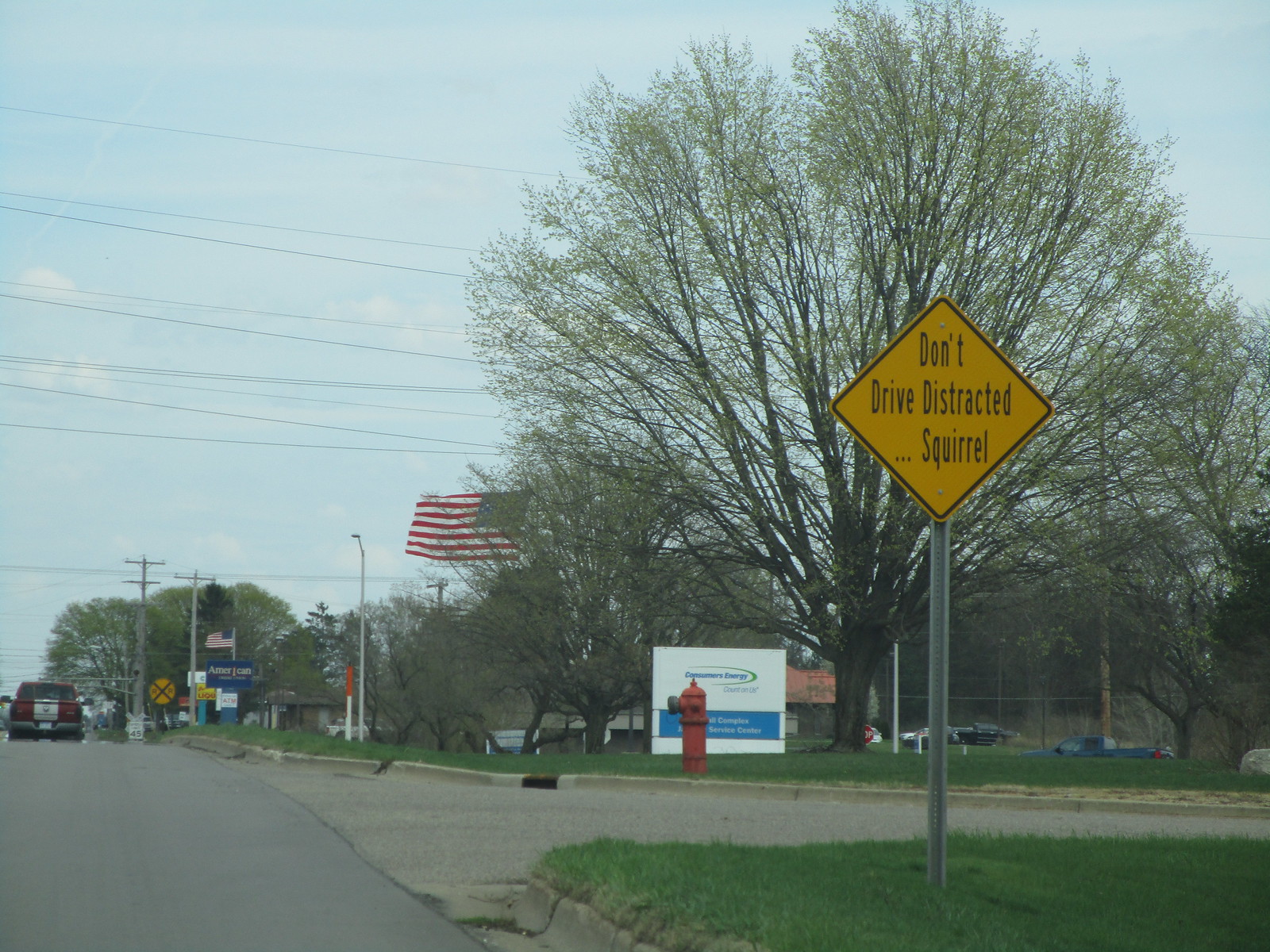In the foreground of the photograph, a gray street stretches across the scene with a strip of green grass bordering it. Prominently positioned on the grass is a metal pole with a yellow sign bearing black text that reads "Don't drive distracted." Beside it, a squirrel is noticeable, adding a touch of wildlife to the urban setting. Behind the pole, a tree with a brown trunk and sparse green leaves stands, its foliage appearing somewhat barren.

In front of the tree, a red fire hydrant is visible, adding a splash of color. Nearby, another sign, blue and white, is mounted in the grass, with an American flag wafting gently in the background. Overhead, power lines cut across a sky that features faint, wispy clouds. Various street signs are scattered throughout the scene, including a speed limit sign and another black and yellow caution sign.

In the background, a red and white pickup truck is parked, next to another American flag. Buildings and cars populate the parking lots, completing this detailed and vivid urban landscape.